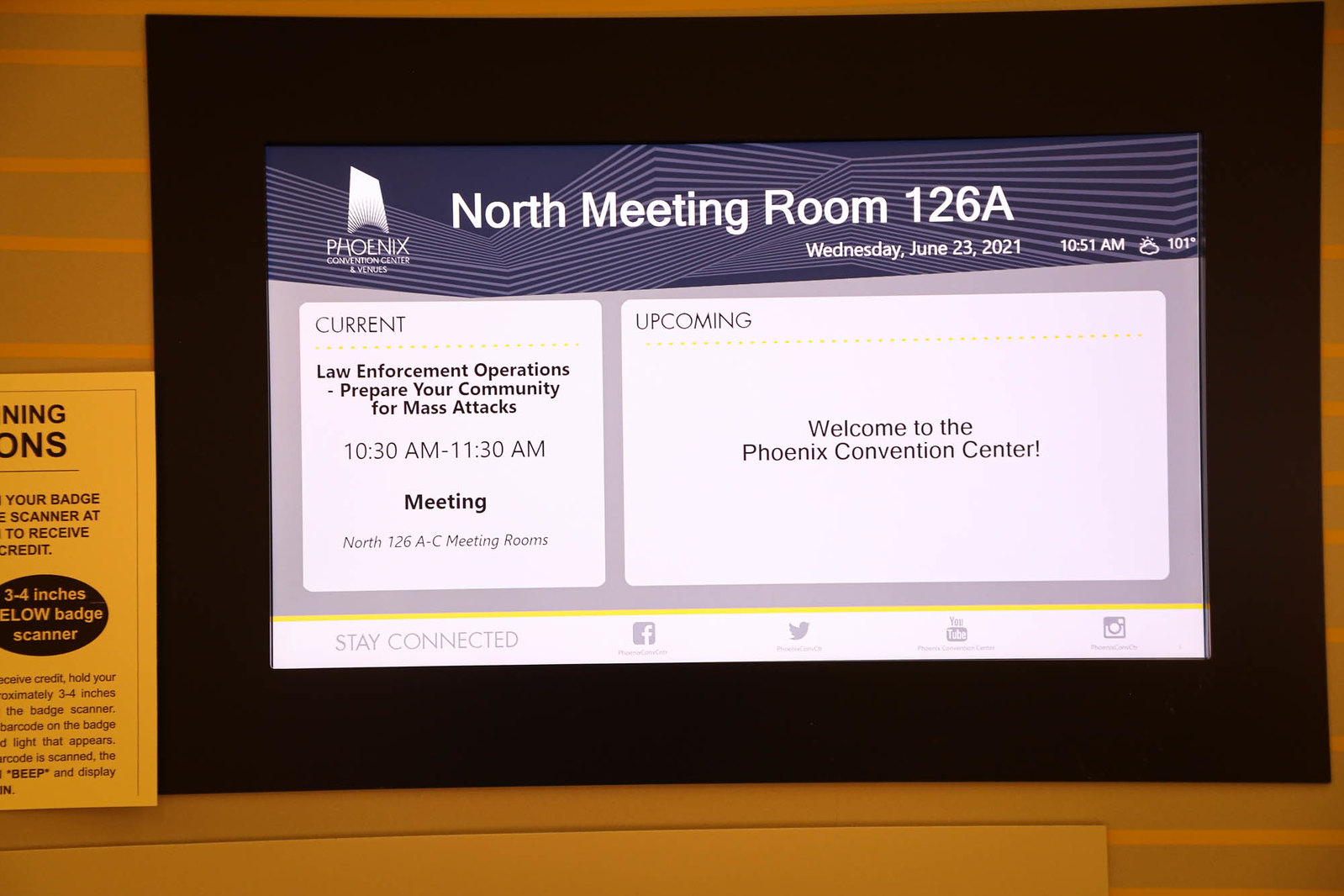The photograph captures a flat screen panel embedded in a wall at the Phoenix Convention Center, showing detailed event information. The top of the screen features the venue identifier "North Meeting Room 126A" along with a timestamp reading "Wednesday, June 23rd, 2021, 10:15 a.m." and an outside temperature of 101°F. Below, the panel displays two sections: "Current" and "Upcoming." The "Current" section announces the event "Law Enforcement Operations: Prepare Your Community for Mass Attacks" scheduled from 10:30 a.m. to 11:30 a.m. in Meeting Room 126A-C. The "Upcoming" section simply welcomes attendees to the Phoenix Convention Center. At the bottom, there is a "Stay Connected" message accompanied by icons for Facebook, Twitter, YouTube, and Instagram. To the left of the screen, there is a yellow poster with partially visible text, likely providing instructions on using a badge scanner for event check-ins, mentioning scanning the barcodes located on badges.